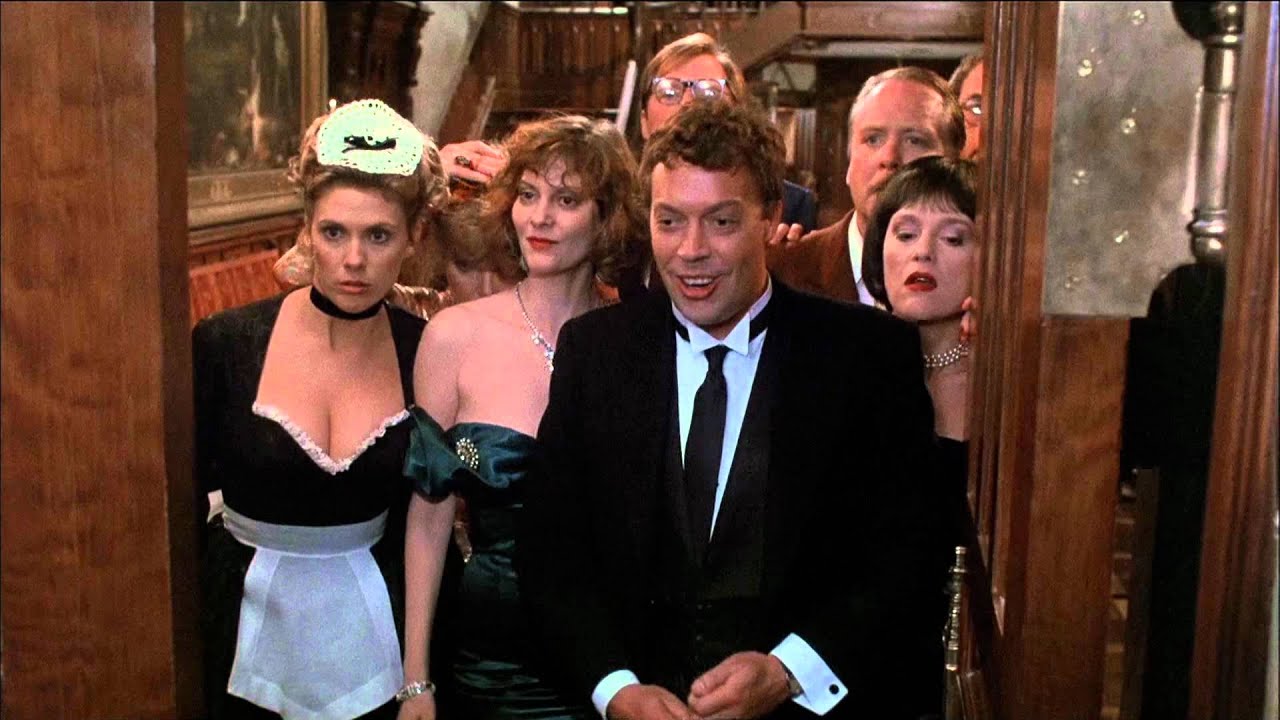The image captures a large group of predominantly well-dressed individuals, likely characters from a movie or television scene, all gathered in what seems to be a wooden room. The setting, while ambiguous, could be likened either to an elevator or the doorway of a train cab, featuring a notable staircase in the background on the left side. Central to the composition is a doorway that appears to be of sliding wooden design, contributing to the room’s predominantly brown and wooden aesthetic. The people are clearly the focal point, all seemingly peeking or entering the space with varied expressions ranging from curiosity to shock. 

In the foreground and to the right is a man wearing a black suit and tie, characterized by his white shirt and broad smile, his brown hair neatly styled. Beside him stands a woman in a low-cut dress, her shoulder-length brown hair framing her face. To their left stands a maid, her ample cleavage visible in her classic black and white outfit, her hair neatly tied up. The other characters crowd behind them, peering over shoulders, adding to the sense of intrigue and suspense in the scene. The colors that dominate the image include shades of brown, black, white, olive, and peach, accentuating the formal and somewhat intimate nature of the scene. A painting or picture is visible on the far left wall, adding to the atmospheric depth of the image.